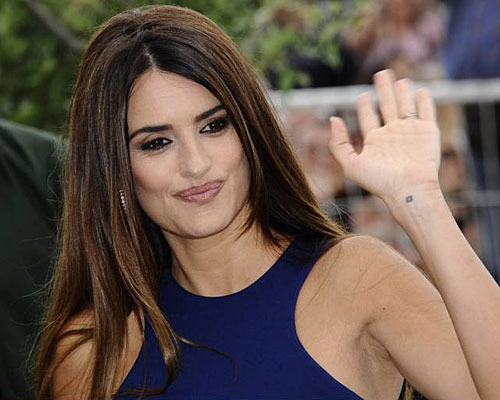A woman, appearing to be in her late 30s or early 40s, is captured mid-wave. She has long brown hair streaked with highlights, and her upraised hand is slightly blurred, indicating motion. A wedding ring adorns her ring finger. She wears a dark blue top that covers her shoulders, possibly part of a dress, though the image is cropped. Notably, a diamond-shaped tattoo is visible on her waving wrist. The background is out of focus, featuring a fence and a few indistinct figures beyond it.